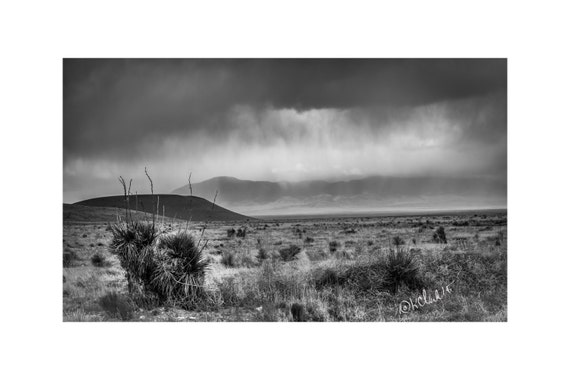A striking black and white photograph captures a desolate desert landscape populated by various dry, bushy shrubs and larger brush in the foreground. The stark scene features scattered, hardy vegetation typical of an arid region, though no cacti are immediately discernible. The horizon showcases two hills to the left - one closer and lighter in shade, and the other more distant and darker. In the background, a larger mountainous area is partially obscured by an ominous, heavily clouded sky. The clouds stretch from left to right, allowing a few sun rays to pierce through, suggesting an approaching storm. The overall tone of the image gives the impression of a sepia or aged effect, contributing to its timeless quality. Notably, the artist's signature, written in cursive, is present at the bottom right corner of the photo, hinting at its authenticity and artistic value.